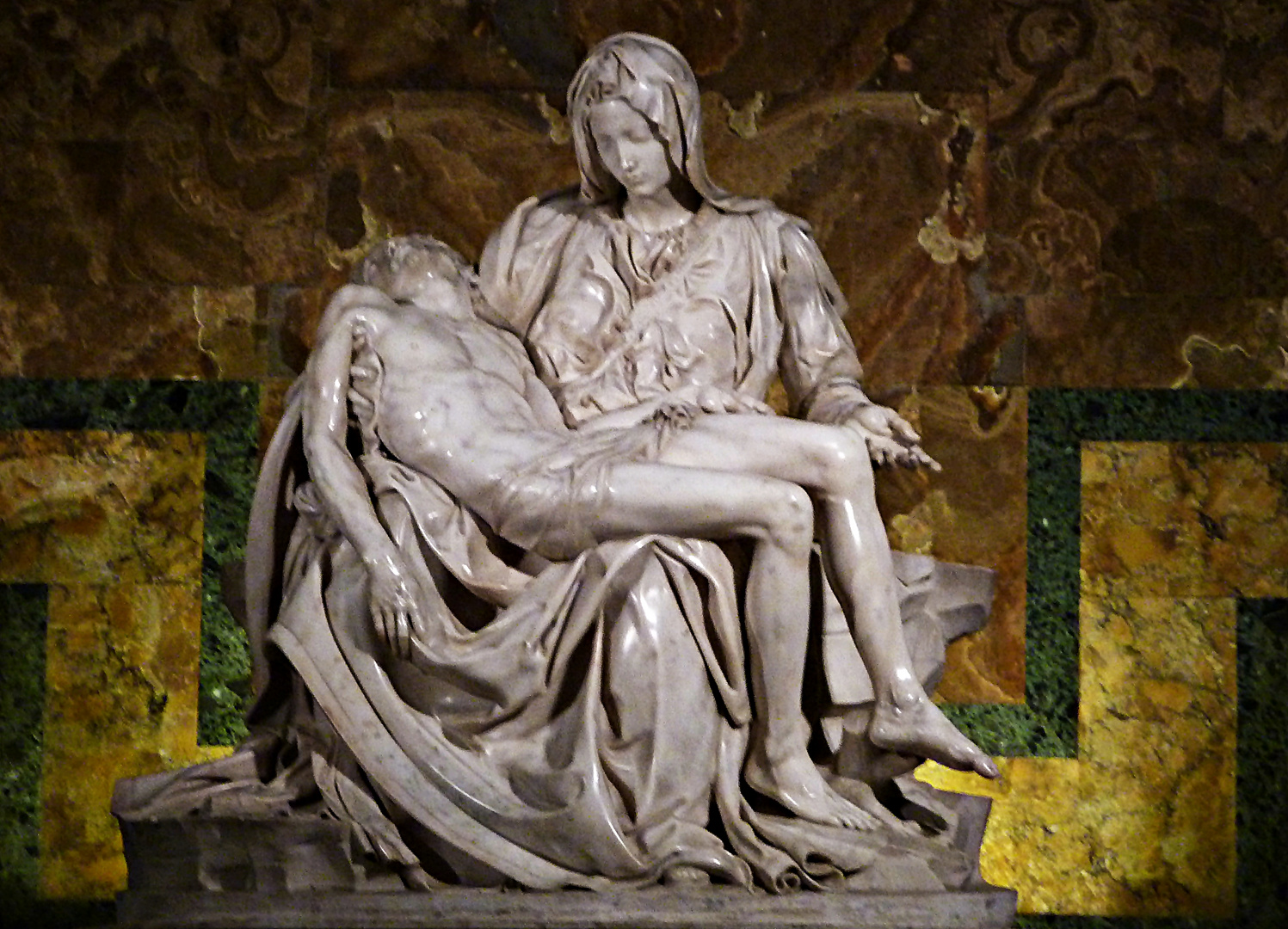The image depicts a grayish-white marble statue, set against a dynamic background of swirled brown and black patterns at the top and a base of horizontally and vertically connected granite-like tiles in lighter and darker brown shades. The statue, slightly blurry in the photo, features a seated woman, robed and hooded, with her head bowed and eyes closed. Her left hand is outstretched with the palm up. She appears to be Mary, holding the bare-chested, dying figure of Jesus, only modestly covered around the waist. Jesus reclines in her lap with his head thrown back, exposing a bearded face, and his right arm hanging loosely beside him. The detailed composition centers on the poignant, tranquil sorrow expressed by the figures, framed naturally by the contrasting background.